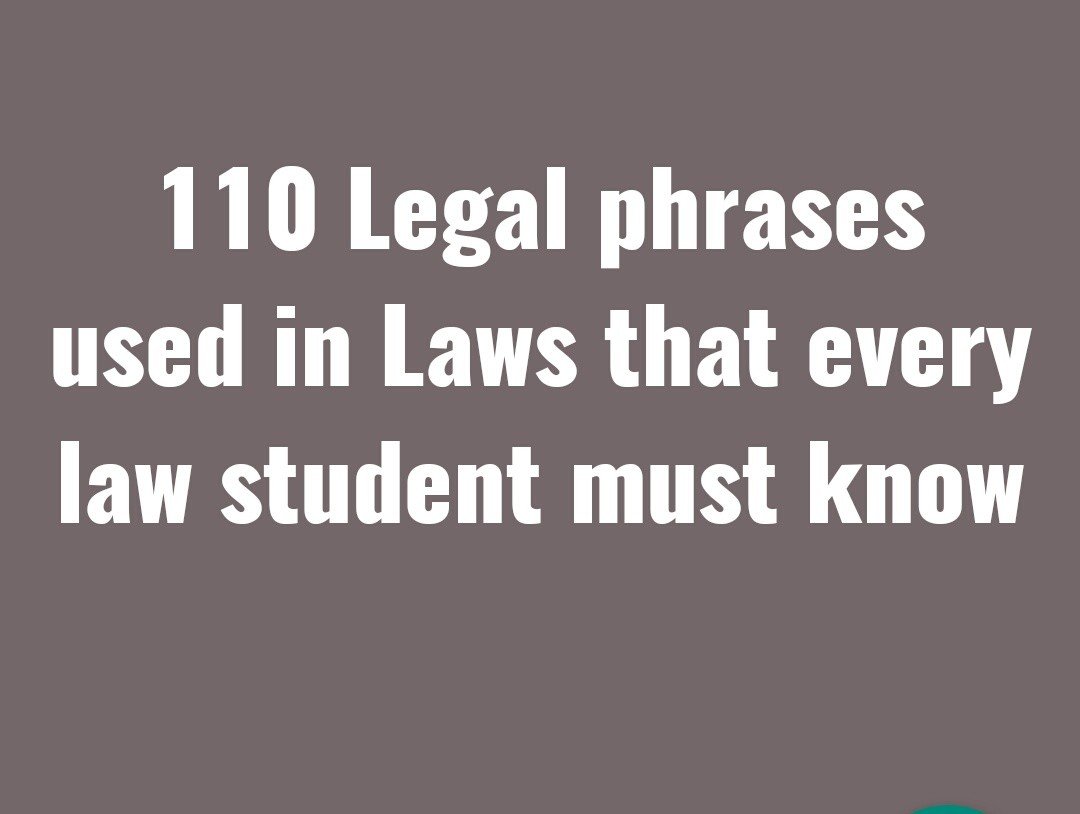The image appears to be an educational slide, possibly from a PowerPoint presentation, featuring prominently white sans-serif text in the center of a grey, mauve background. The text is organized into three lines: "110 legal phrases," with the word "legal" capitalized, followed by "used in laws," with "laws" also capitalized, and concluding with "that every law student must know." Notably, the numbers and first letters "L" in "legal" and "laws" are capitalized, while the rest of the text remains in lowercase. The number "110" is written in numerals. Additionally, the font used is reminiscent of Arial, with no serifs and a distinctive styling on the letter "G." At the bottom right corner of the image, there is a small green circular element. This slide is likely introductory material aimed at law students, designed to present essential legal phrases used within legal texts.